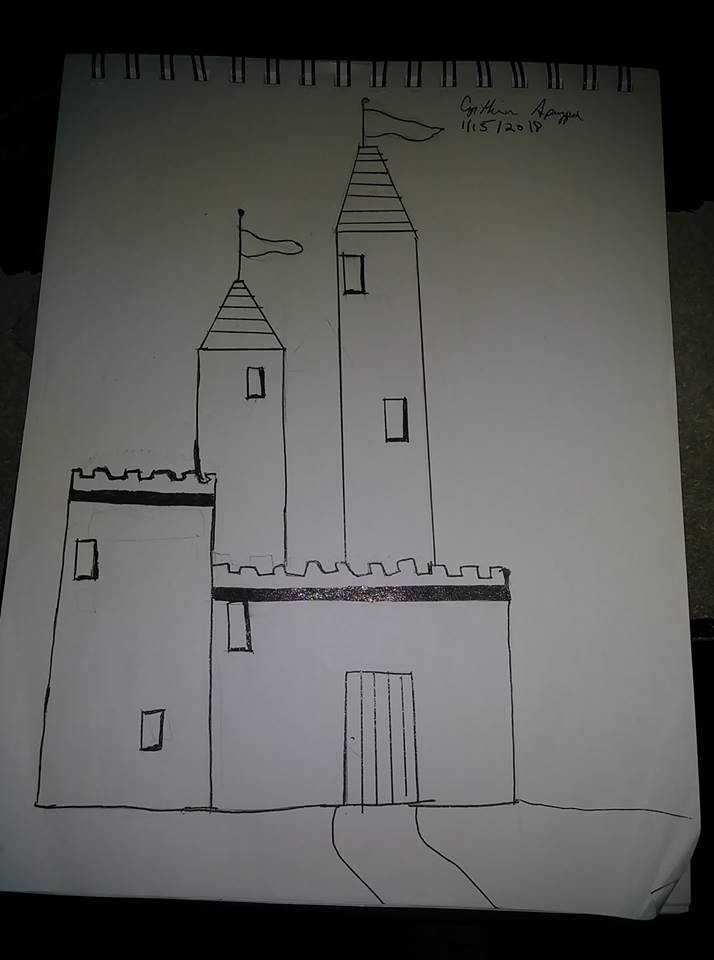This image depicts a child's drawing from an art class, preserved in a white spiral-bound sketchbook. At the top of the page, the name "Cynthia Apagu" (though the last name is uncertain) is written in cursive. The drawing is dated and signed in the upper left corner, with a date of January 15th, 2018.

The central focus of the drawing is a castle set against a simplistic landscape. The artist has drawn a horizontal line to represent the ground, which runs continuously beneath the castle structure. A path extends from the foreground up to the castle's entrance. 

The base of the castle is a prominent rectangle, characterized by crenellations along the top, creating a series of up-and-down battlements. To the right side of the castle, a turret has been illustrated, featuring two small windows and matching crenellations.

Behind the main rectangular building, two towers rise with peaked roofs adorned with flags. Of these towers, the left-hand one is taller and features a window midway up on the left side and another in the top right corner. The shorter tower on the right has a single window positioned in the upper left corner.

The detail and imagination displayed in this drawing reflect the developmental artistry typical in children’s art, offering a charming and medieval-themed scene.